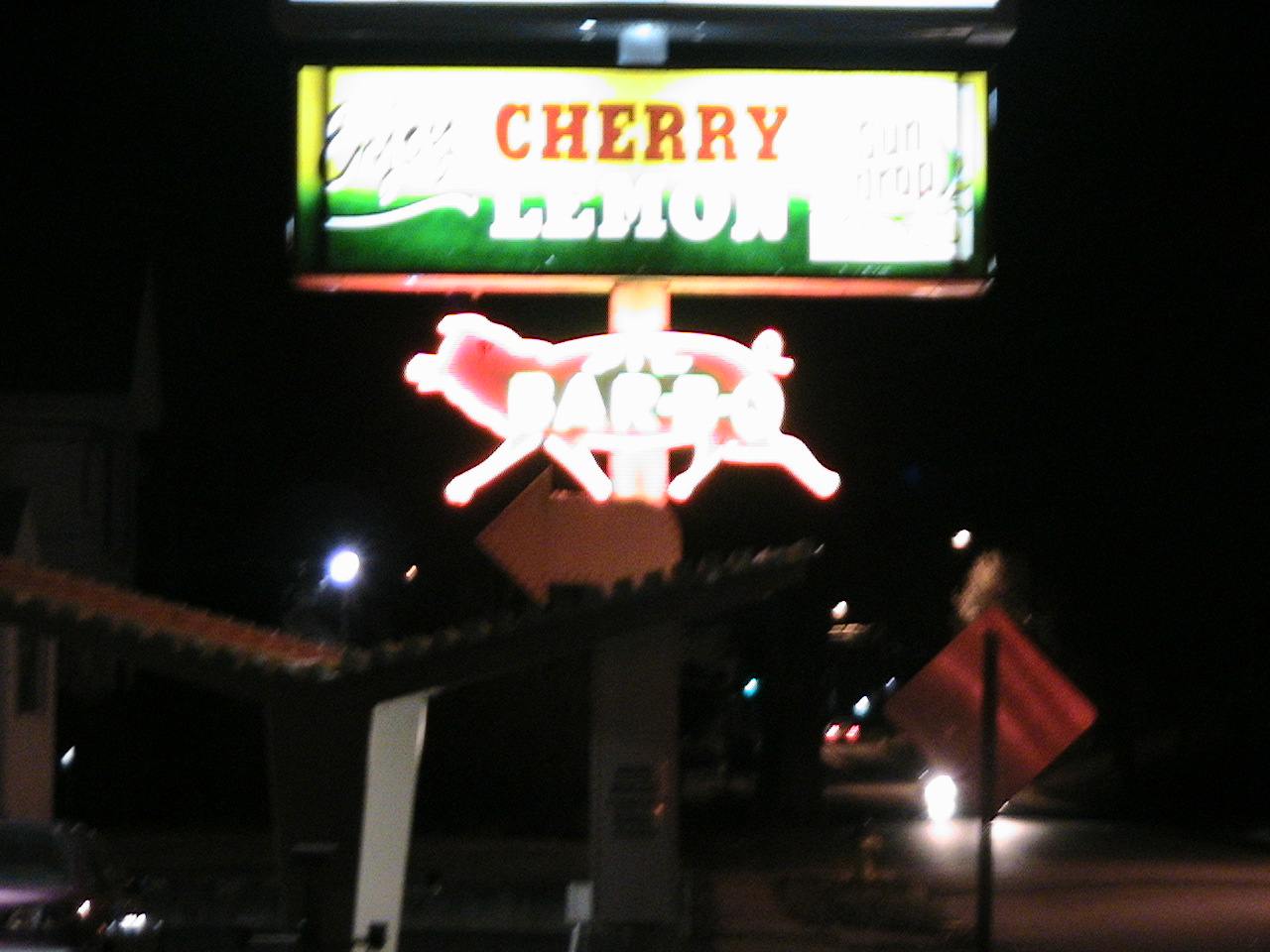This nighttime photograph captures a blurry, neon-lit sign for a barbecue restaurant. The sign itself is a horizontally oriented rectangle mounted on a single pole, glowing brightly against the dark background. The top portion of the sign, lit with bright white light, is difficult to discern due to its poor exposure. However, in bold red capital letters, the name "CHERRY" is visible, with the word "LEMON" in white text beneath it. The bottom third of the sign has a green hue, and the edges appear to have a yellowish tint, though it's challenging to see clearly. Below this rectangular sign, there is a glowing pink neon outline of a pig walking left, with "BAR-B-Q" illuminated in white text inside the pig's body. The scene includes a car with its headlights on, approaching from the right side of the image, highlighting the sign's roadside location.